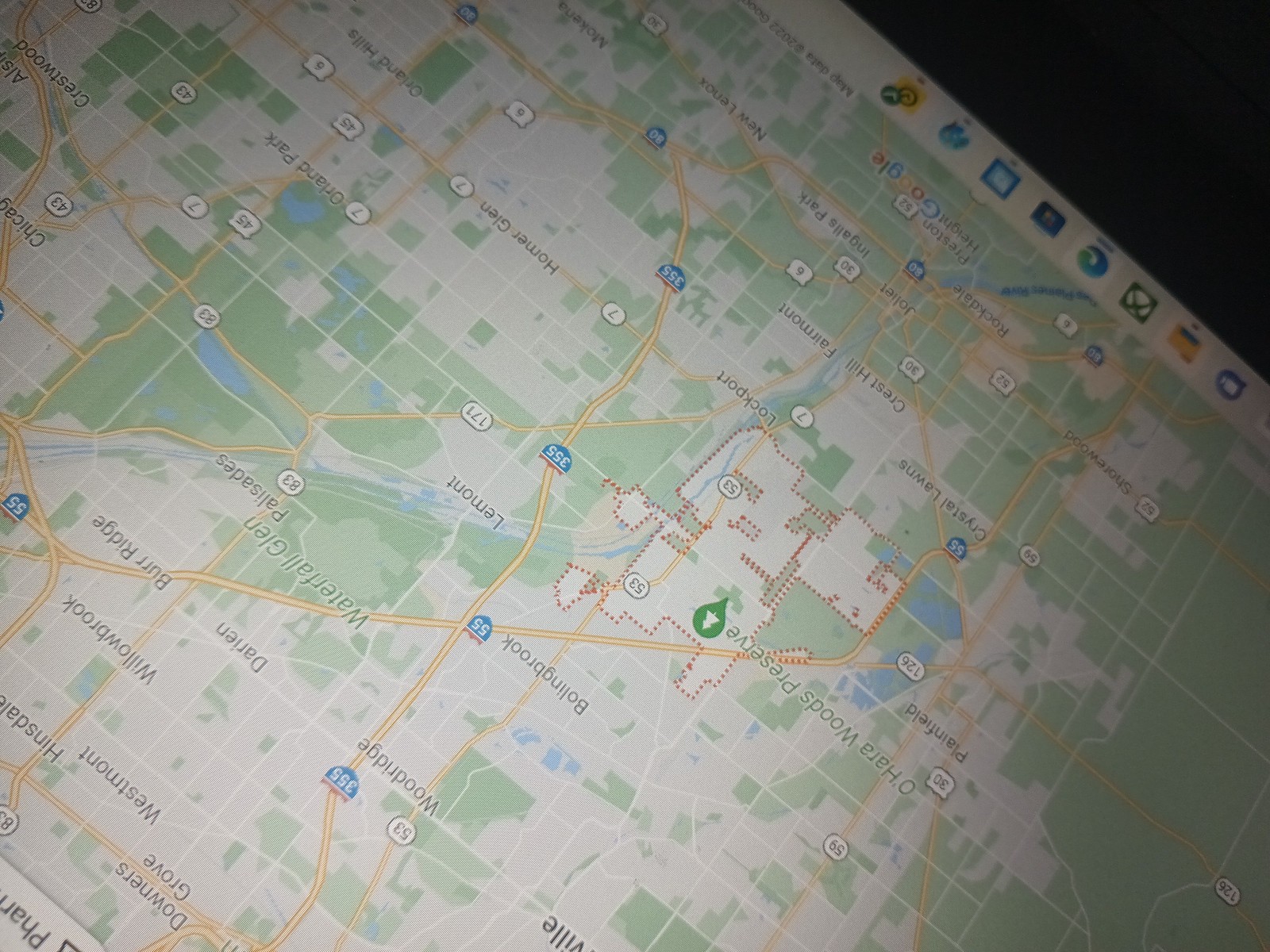This photograph captures an upside-down screenshot of a map displayed on a laptop screen, featuring the detailed layout of a city with various marked streets, neighborhoods, parks, and water bodies. Despite its inverted orientation, the text on the map is still legible, revealing notable locations such as O'Hara Woods Preserve and Bowling Brook. Prominent areas like Woodbridge and Darien are also labeled. Major thoroughfares include I-355 and I-55, along with routes I-83 and I-171. A distinct park, identified as Waterfall Glen Palisades, is visible. The presence of icons at the top of the screen suggests the image is indeed taken from a computer or laptop interface. All these elements combined help to deduce the city being referenced in this map.